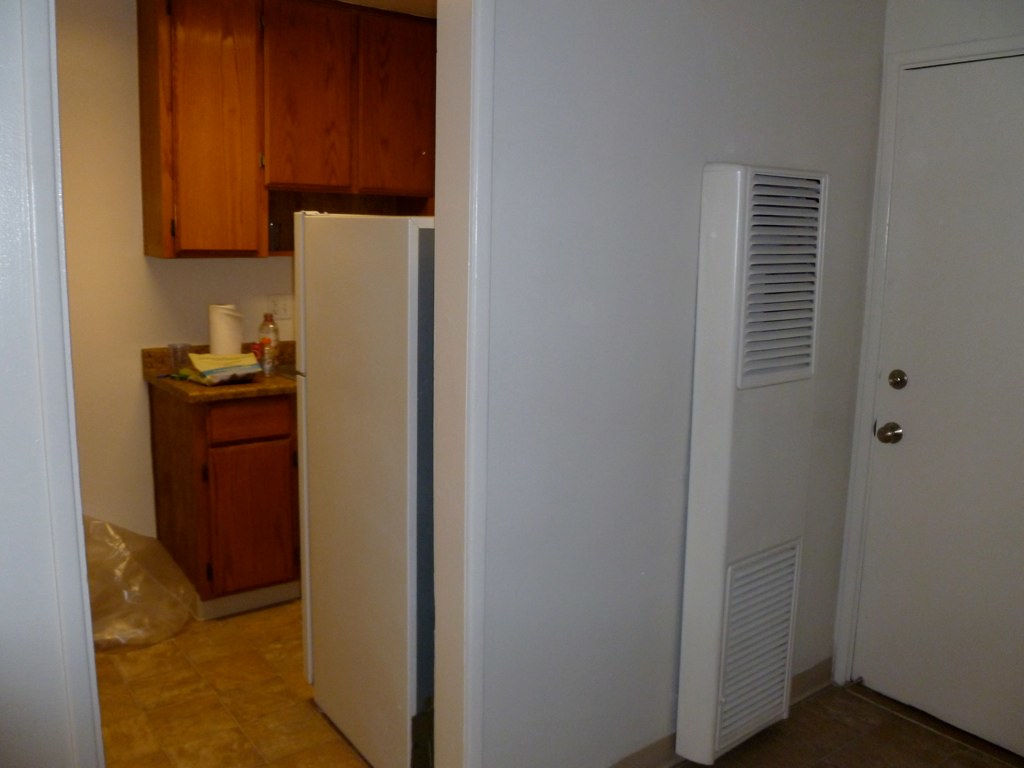This image depicts the entryway of a compact studio apartment. On the right side of the entrance, there's a white door equipped with a silver handle and a silver deadbolt lock. Adjacent to the door is a white wall featuring an HVAC vent with slats on both its top and bottom sections. As you proceed further into the room, you encounter a small kitchenette. Immediately visible is the side of a white refrigerator. Opposite the refrigerator, there's a set of dark mahogany cabinets, consisting of one elongated cabinet flanked by two shorter ones. Below the cabinets is a counter, on which a roll of white paper towels is placed. The flooring throughout this space is an aged brown linoleum, and notably, a brown towel is lying on the floor near the cabinetry.